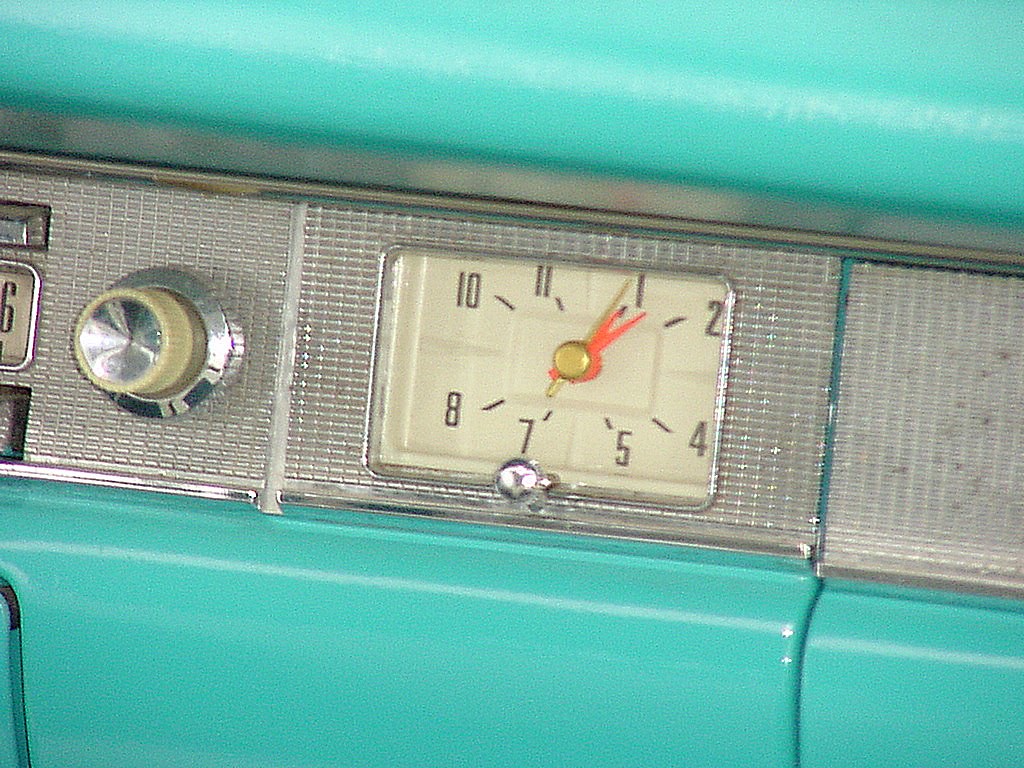This photograph captures the interior of a vintage 1950s classic car, featuring a striking turquoise green dashboard. The centerpiece is an elegant clock with a tannish-yellow background and bold, block numbers. The clock's orange hour and minute hands, alongside a slender gold second hand, display the time as approximately 10 past 1. Adjacent to the clock on the left is a nostalgic turn-dial radio, harking back to an era when finding a station required a manual twist rather than a simple button press. The detailed elements and rich colors evoke a sense of timeless charm and retro sophistication.